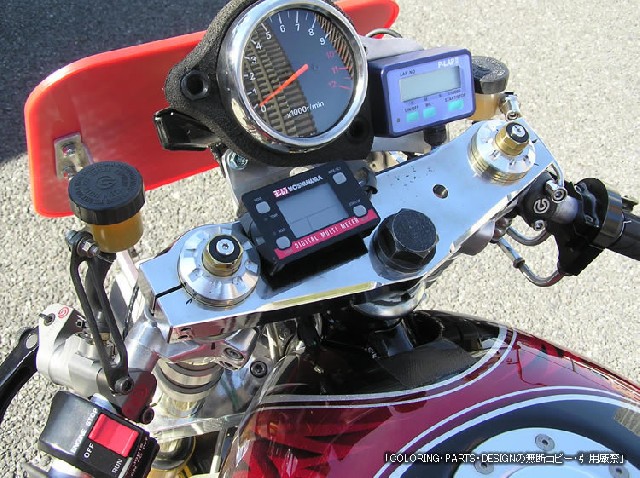The image showcases the front section of a motorcycle with a focus on its dashboard and handlebars. Central to the image is a black-faced odometer with numerals ranging from 0 to 12; the numbers 0 to 9 are white, whereas 10, 11, and 12 are distinguished in red. Adjacent to the odometer are additional meters: one black meter featuring a screen with four buttons, and another light purple meter with a screen and three buttons. The motorcycle's frame is predominantly red with black accents, accompanied by a mix of black and silver handlebars. There are also small containers likely designed for holding various fluids. A notable feature on the bottom left is a red button labeled "OFF" or "TEF," and on the bottom right, text reads “coloring parts design,” followed by Chinese characters.